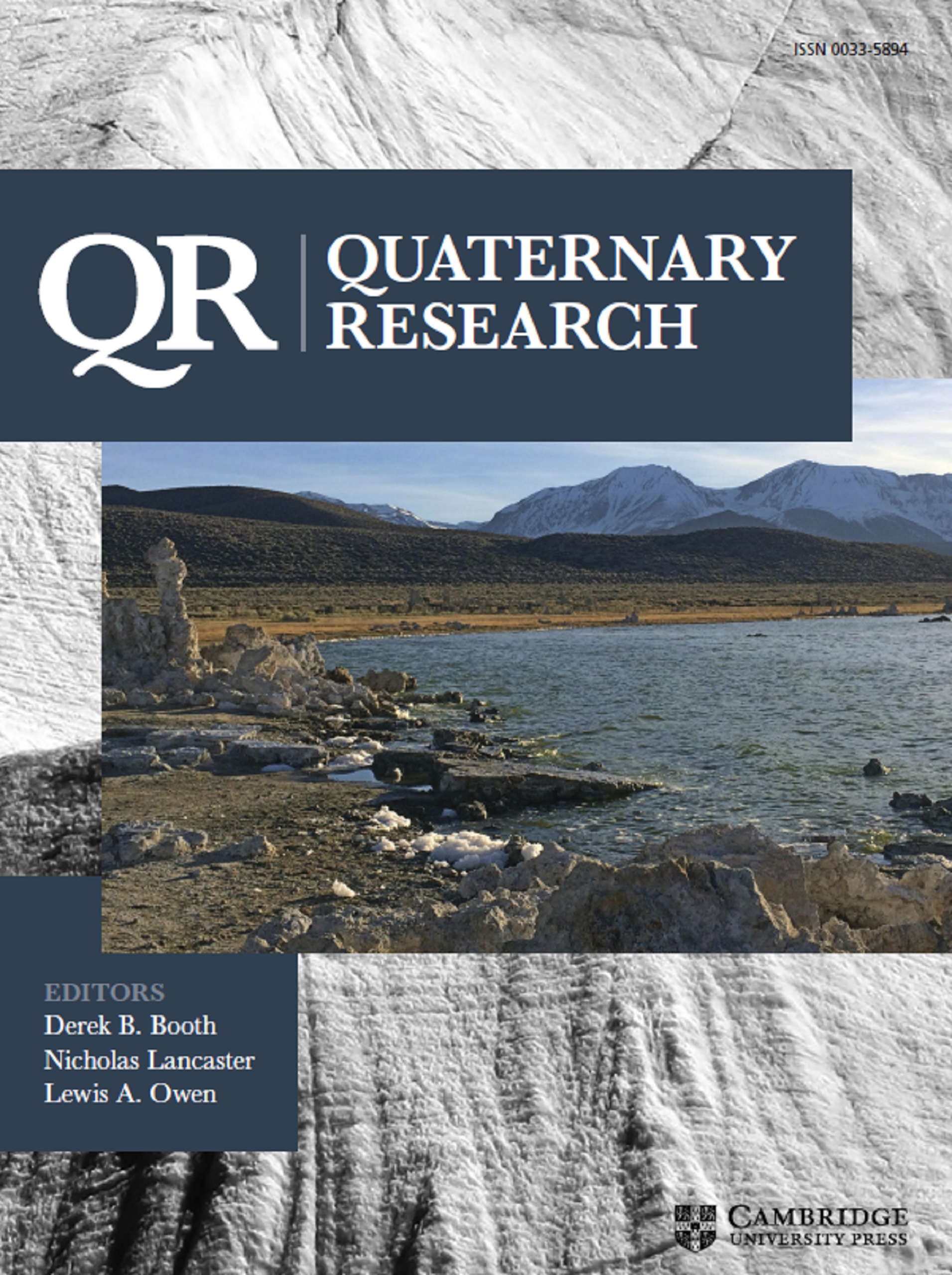This image depicts the cover of QR, Quaternary Research, published by Cambridge University Press. The top section prominently features the title "Quaternary Research" and a giant "QR" in white text against a black rectangular background. Below the title, centered on the cover, is a photograph of a serene lake surrounded by rocky terrain, with snow-covered mountains in the distance. The vibrant blue of the lake contrasts beautifully with the gray and white tones of the mountains and rocks. The editors' names, Derek Booth, Nicholas Lancaster, and Lewis A. Owen, are noted towards the bottom left. The Cambridge University Press logo is positioned at the bottom right of the cover. The overall color scheme of the cover is primarily gray, with white text providing a clean and professional appearance.